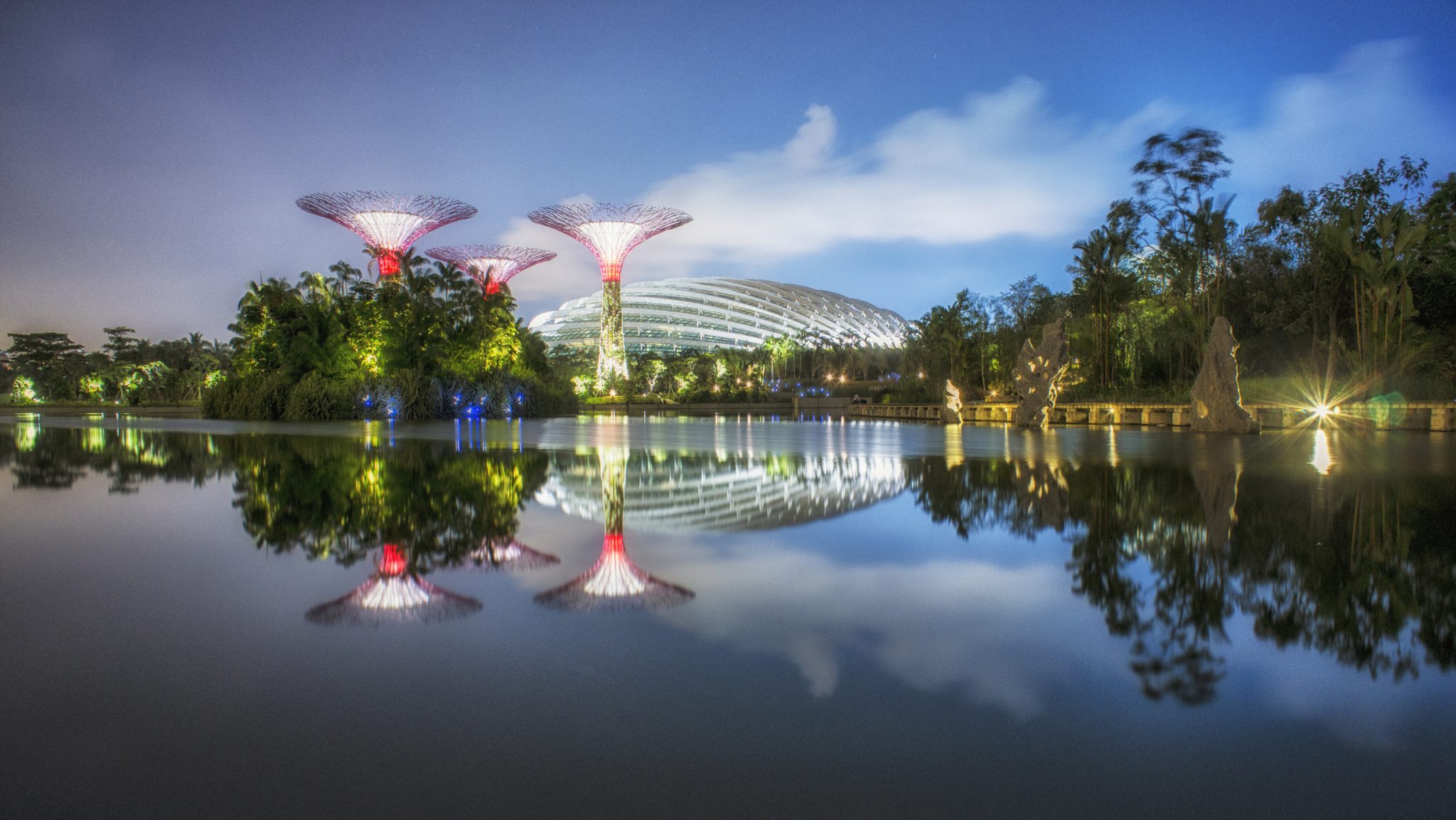In this landscape-oriented photograph, we observe a tranquil waterscape featuring a mirror-like, perfectly still body of water in the foreground that reflects the entire scene above. Dominating the background is a striking modern stadium complex, identifiable by its towering white dome with numerous clear windows. This stadium, reminiscent of a World's Fair or Olympic venue, is flanked by an array of lush greenery, including palm trees forming a jungle-like setting along the horizon.

Positioned prominently in front of the stadium are three distinctive, illuminated towers with shapes reminiscent of wine or martini glasses. These towers exhibit a gradient of lights from green at their bases to red and purple towards their tops, culminating in bulb-like yellow fixtures. Additionally, another set of purplish lights is visible just in front of the stadium. Adding to the scenic complexity, sculptures or rock formations are strategically placed near the water's edge, further enriching the view. Above this serene yet striking tableau, the sky is adorned with calm blue clouds, completing the picturesque and dramatic symmetry of the photograph.